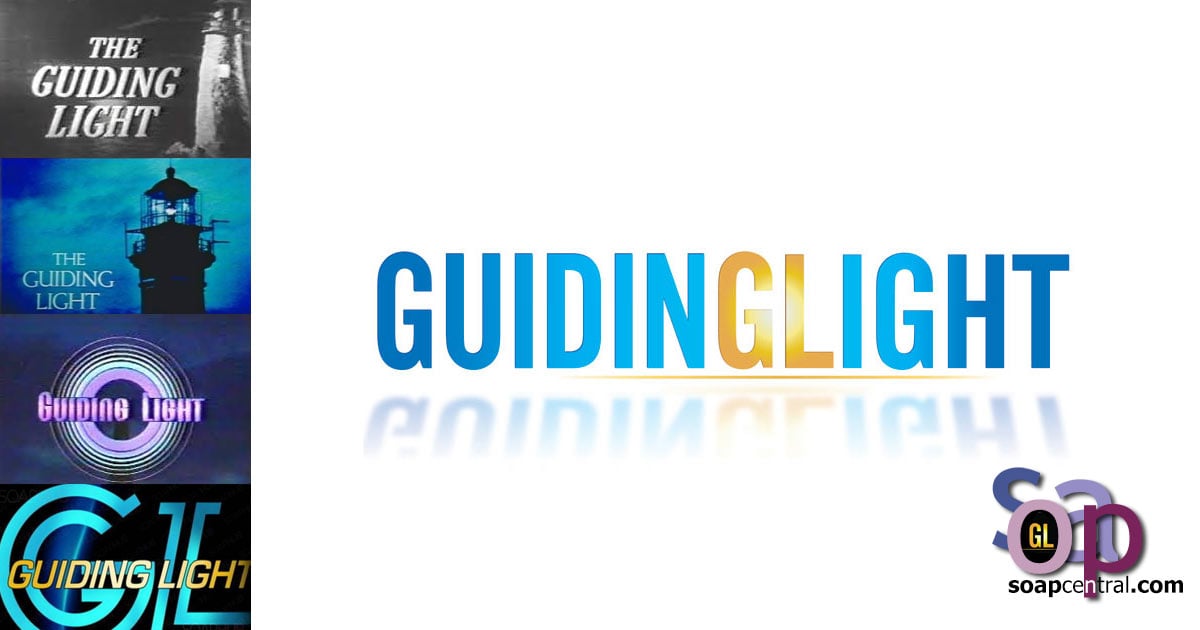This detailed advertisement for the television soap opera "Guiding Light" prominently displays the show's evolving branding over time. On the left side, a column of four images showcases various logos from the show's history, starting with the earliest logo at the top and progressing to more modern iterations below. In the center, the name "Guiding Light" is boldly featured in large, dark blue font, with distinct accents where the second "G" and the first "L" are highlighted in gold. Below the main title, there's a mirrored reflection of the text, adding a graphic illusion to the white background. The bottom right corner features the SoapCentral.com logo, indicating that the advertisement is from SoapCentral, a website dedicated to TV soap operas, with specific emphasis on "Guiding Light."